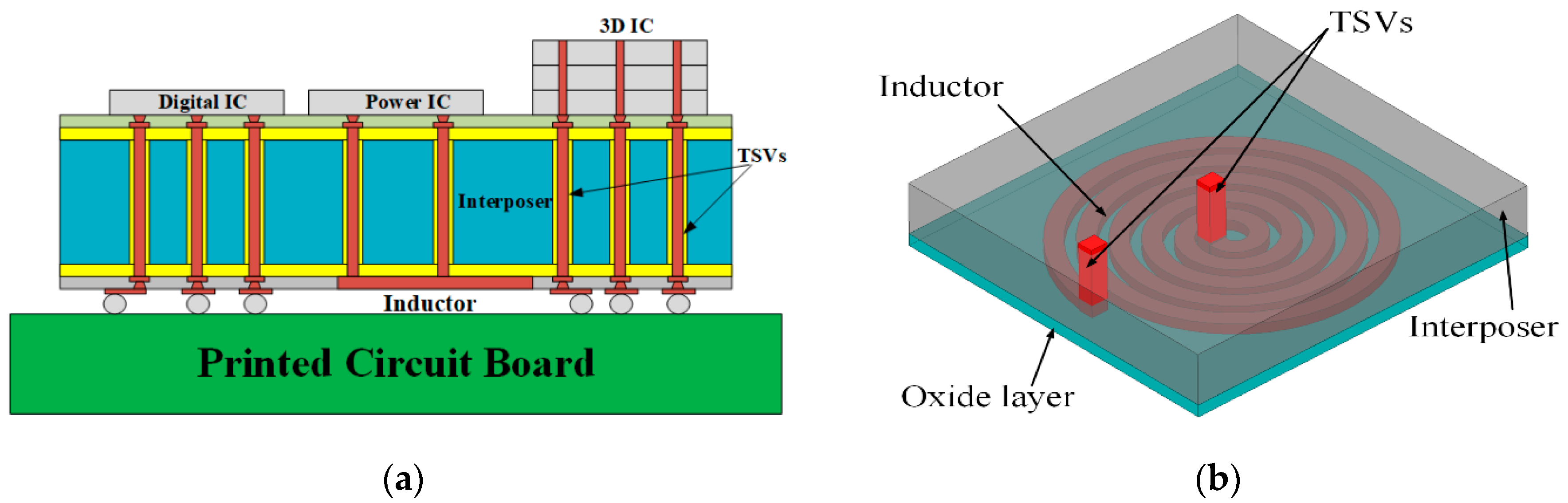The image consists of two detailed diagrams side-by-side, both related to a printed circuit board. On the left, labeled "A" and identified in a green box as "Printed Circuit Board," the diagram showcases various components, including a digital IC, power IC, 3D IC, TSVs, an interposer, and an inductor. The visual elements include a large horizontal blue line bordered by two smaller yellow lines, with eight vertical red lines interspersed, and multiple blue and gray rectangles. These components are intricately layered and labeled, though the text is small and somewhat difficult to read.

On the right, a zoomed-in view provides a closer examination of key components such as the inductor, TSVs, interposer, and oxide layer. This section is labeled with the terms "inductor," "TSVs," "interposer," and "oxide layer," offering a deeper understanding of the internal structure. It depicts a large rectangular prism—resembling the dimensions of a pizza box—with a red coil inside, flanked by two touching rectangular prisms. The detailed labels and specific highlighting of these elements provide a comprehensive look at the printed circuit board’s organization and function.